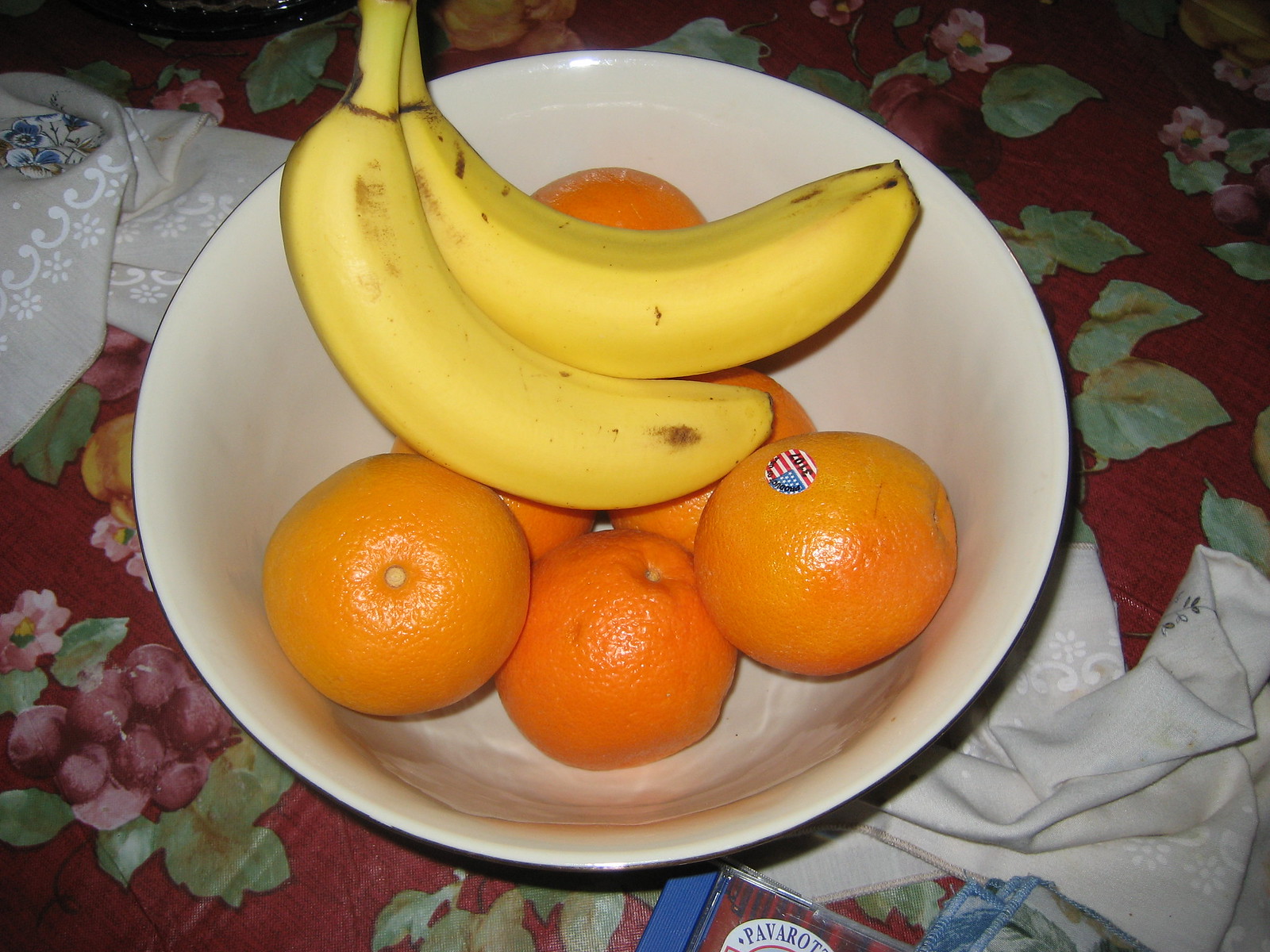This still life color photograph captures a top-down view of a bowl of fruit, exuding a charming and homey atmosphere. The bowl, which could be ceramic or glossy plastic, features a white interior with a possibly shadowed dark rim. It cradles six vibrant oranges at the bottom, one of which has an American flag label with the item number 3102, providing a touch of everyday authenticity. Resting atop the oranges are two not-quite-ripe bananas, adding a vertical contrast to the composition.

The bowl sits on a richly burgundy tablecloth adorned with an intricate design of pink flowers with yellow centers, green leaves, and what appears to be grape clusters, lending a burst of color and pattern to the scene. Positioned just outside the bowl, at the top left and bottom right of the photo, are partially folded cloth napkins or bandanas in a tan or light gray hue with a classic white bandana design. Adding an unexpected musical element to the tableau, the top edge of a Luciano Pavarotti CD in a jewel case peeks into the bottom right corner of the frame, its bold lettering partially visible: "P-A-V-A-R-O-T...". This detail infuses the image with a subtle cultural note, marrying food and music in a casual yet elegant setting.